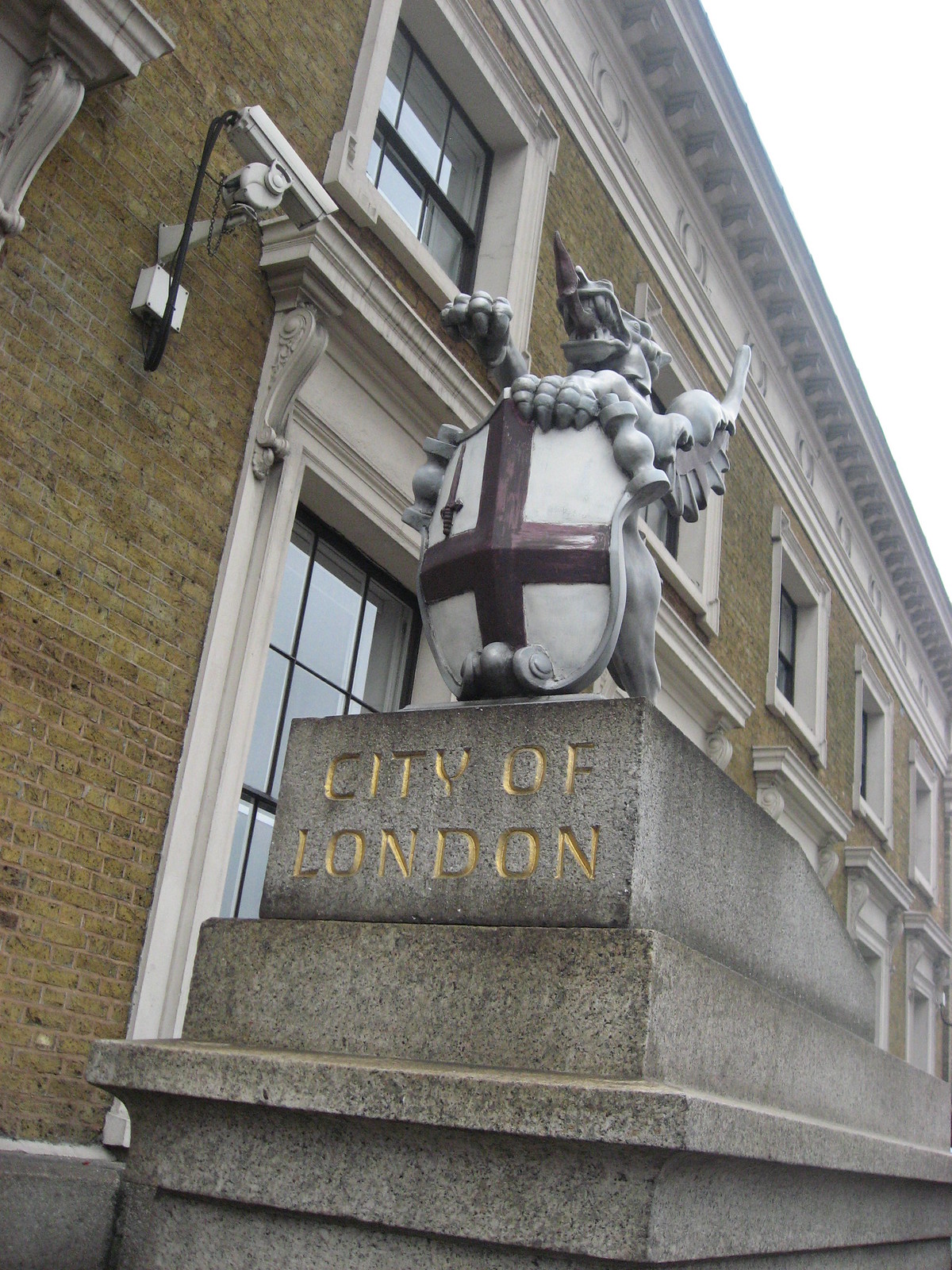In this detailed photograph, we see a dramatic statue prominently displayed on a concrete platform. The platform has the words "City of London" carved and painted in yellow on the top plaque, set against a regular grey concrete backdrop. The statue itself resembles a dragon with sharp teeth, a jagged horn, and wings extending majestically behind its back towards the sky. The dragon's right hand grasps a curved shield featuring the England flag design and a small sword in its top left quadrant, while its other hand is raised. Only the back leg of the dragon on the right side is visible, as its left leg is obscured. Below the base, there are three layered plaques: the top, largest one with "City of London" inscribed, and two wider, thinner plaques beneath it.

Adjacent to the statue, on the left, is at least a two-story building with dark brown brick walls. The windows of this building are sectioned into grids of nine or twelve panes by thin black bars. Between the first and second floor windows, a CCTV camera is mounted, facing towards the statue. The overall scene captures a blend of historical symbolism and urban surveillance, set against the backdrop of the city’s architecture.